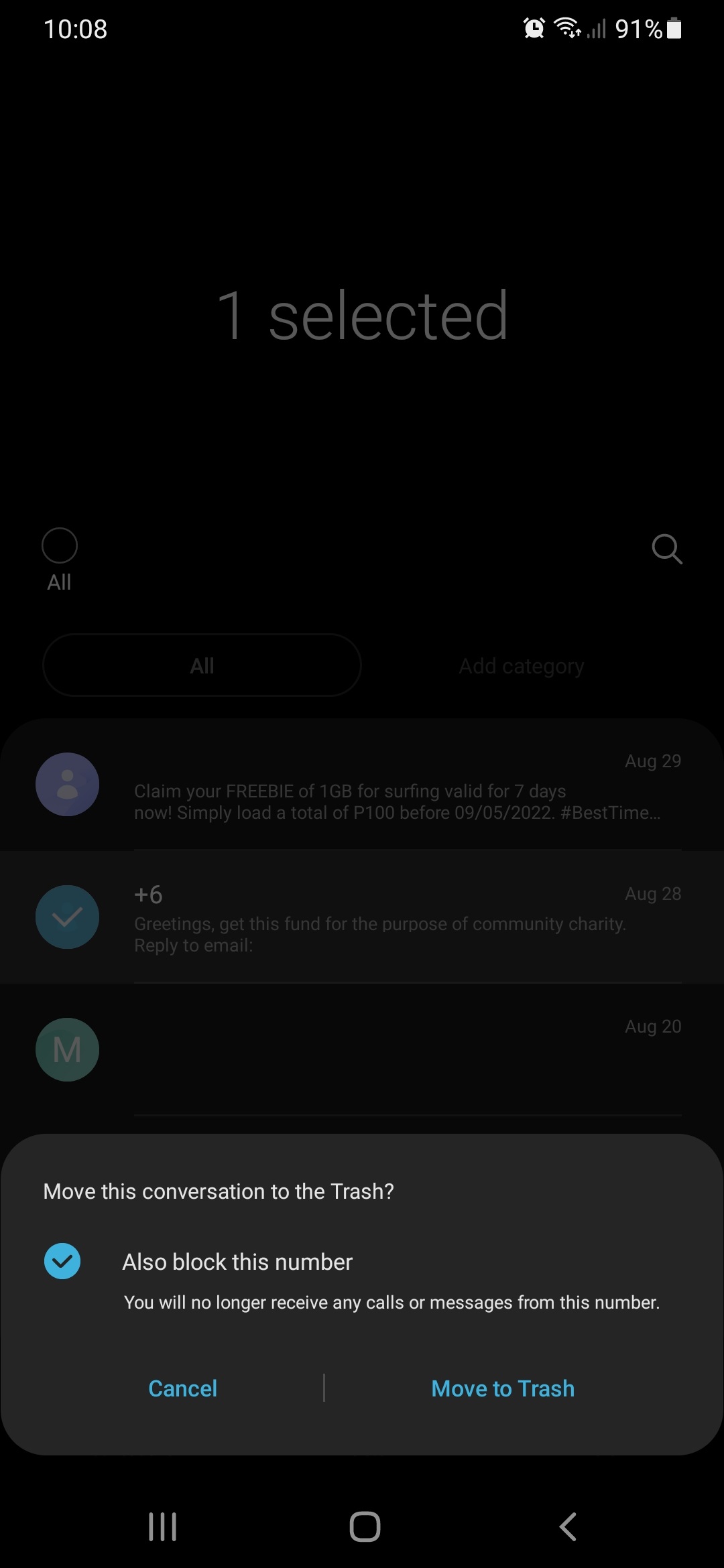This is a detailed screenshot of the settings section of a mobile phone. The time displayed in the top left corner is 10:08, while the battery level is shown as 91% with a battery icon in the top right corner. The background is black, and prominently in the middle of the screen, large white text reads "One Selected." 

On the same row, to the left is an 'All' bubble, and to the right is a magnifying glass icon. The interface features two tabs: 'All' and 'Add Category,' with 'All' currently selected. 

Three rows of messages are visible. The first row reads, "Claim your freebie of one gigabyte for surfing valid for seven days" and is dated August 29. The second row is titled "Greetings. Get this fund for the purpose of community charity" and is dated August 28. Notably, this row includes a "+6" at the top, possibly indicating additional unread messages. The third row, although without a message, is dated August 20.

A pop-up bubble at the bottom of the screenshot indicates actions for handling selected messages. It says, "Move this conversation to the trash," accompanied by a blue checkmark. To the right of the checkmark is an option to "Also block this number." Below these options, there are two buttons: a 'Cancel' button on the left side, and a 'Move to Trash' button on the right, both in blue.